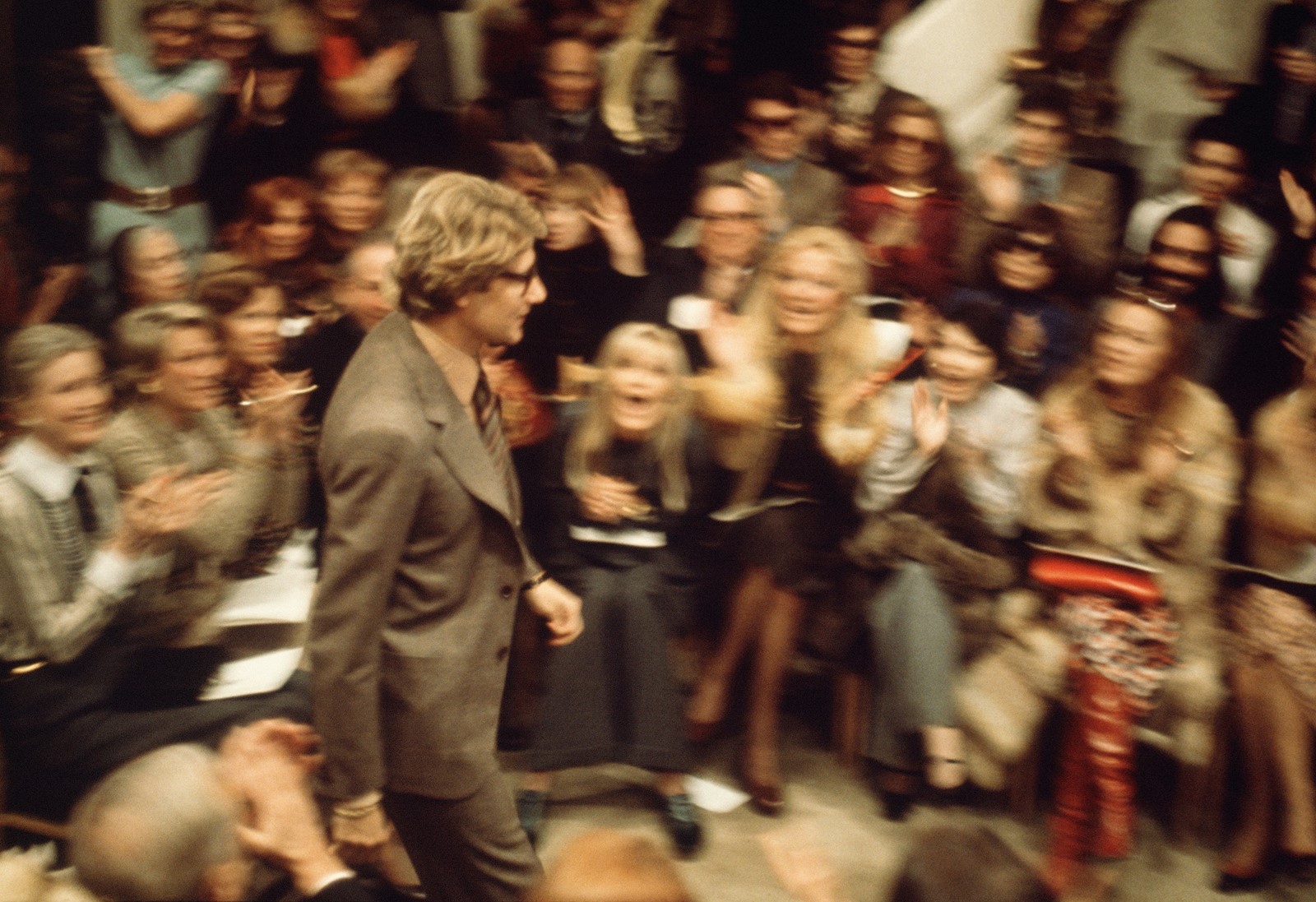This photograph captures a distinguished moment from a fashion show, likely featuring the iconic fashion designer Yves Saint Laurent. The man in the image, identified by many as Yves, is confidently walking down the runway in a well-tailored tan suit complemented by a tan button-up shirt, a striped brown tie, a bracelet, and a watch. His distinctive look is completed with dark tortoise shell glasses and wavy brown hair that elegantly frames his face and touches his ears.

The scene is vibrant with an audience filled with elegantly dressed women and men, standing or seated in rows on either side of the aisle, all showing their admiration with enthusiastic clapping. The front row is notably populated with women who seem enthralled and possibly starstruck, with one observer noting a likeness to Liza Minnelli among them. The excitement is palpable as some women lean forward with open mouths, dressed in black and white outfits, clapping vigorously. The background blurs slightly, but it's noticeable that aside from the seated spectators, a few individuals stand in the further rows, enhancing the lively, almost electric atmosphere of the show.